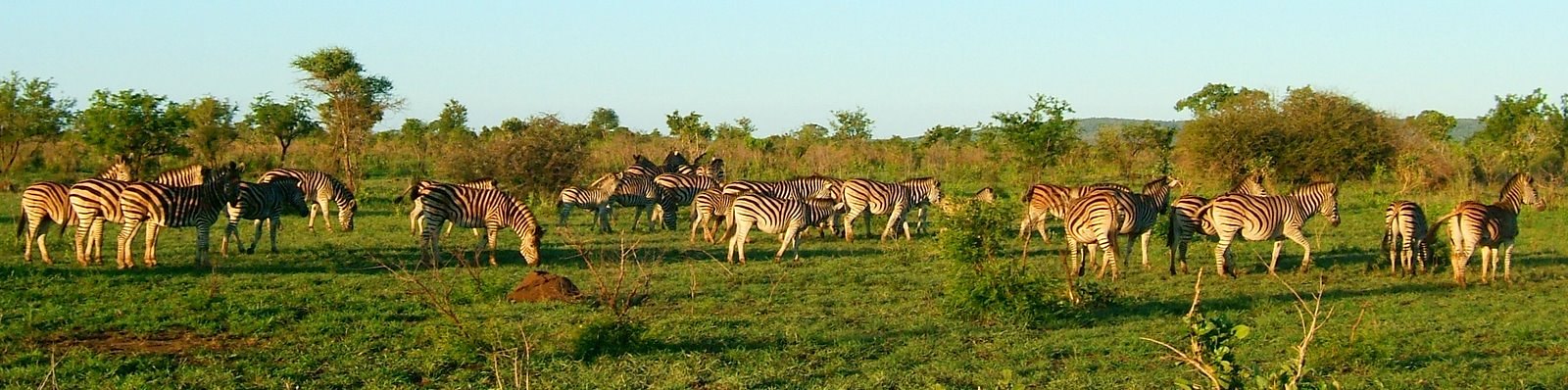A panoramic photo captures a vibrant African savannah teeming with life under a clear, bright blue sky. The wide, yet narrow frame showcases around 20 zebras, all grazing peacefully in lush, green grass that stretches across the entire plain. Scattered bushes dot the foreground, while the background features an array of trees, some lush with various shades of green leaves and others showing signs of drying with browns and tans. The zebras, predominantly black and white, appear to vary in age, with a mix of adults and some younger ones. Reflections of the sun give a few of them a slightly brownish hue. Mounds of dirt are visible among the herd, adding to the natural, undisturbed look of their habitat. The scene exudes tranquility as the zebras roam and graze in their natural environment.